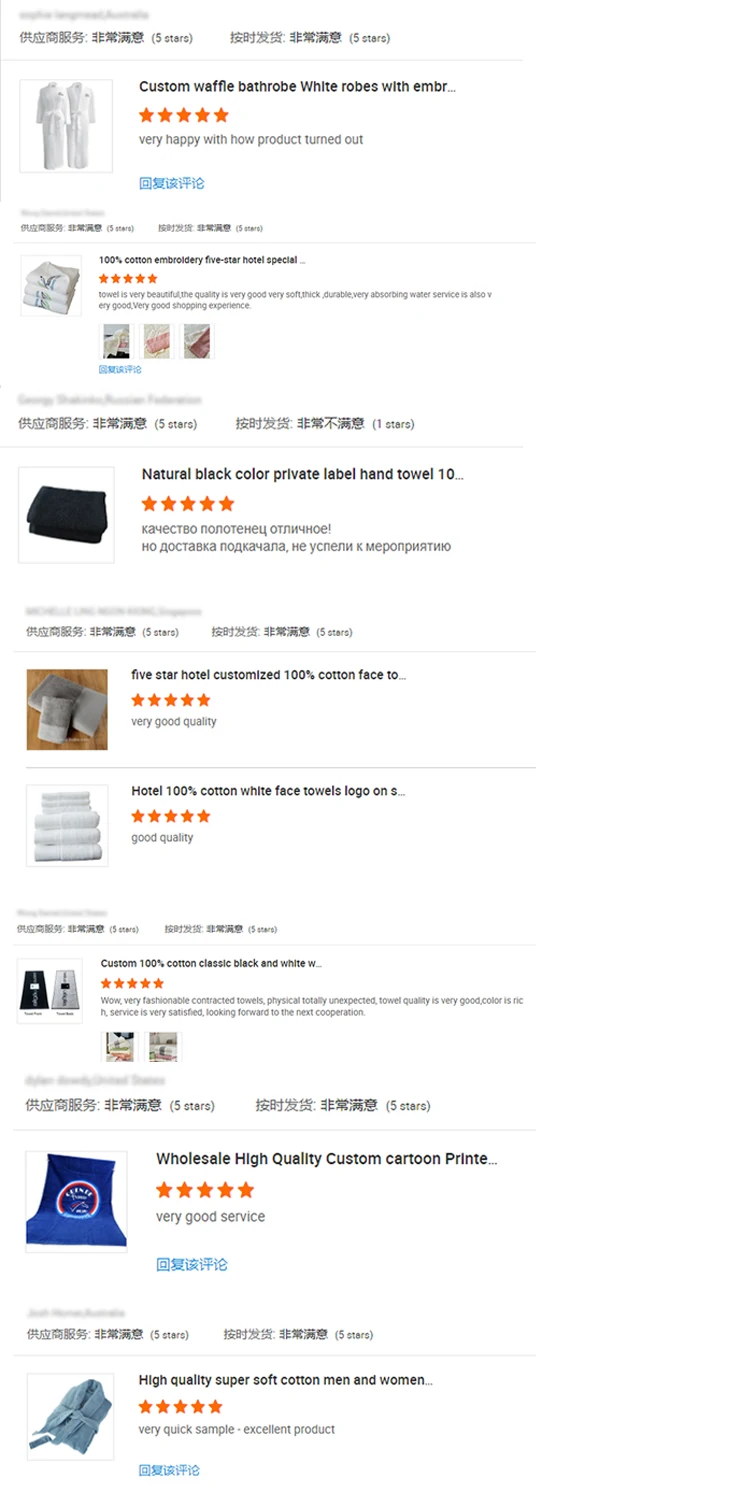**Caption for Image Review Page:**

The image displays a review page with three distinct product reviews, each set within a rectangular area bordered by light gray lines. 

1. The first review showcases two plush white bathrobes, set against a light gray border. On the right side, a bold black header reads, "Custom Warm Bathrobes, White Robes with AMBR or EMBR...". Due to pixelation, the full text is difficult to discern. Below the header, a five-star rating is prominently displayed, with the stars filled in orange. A gray, non-bold font below the stars reads, "Very happy with how product turned out." Beneath this line of text lies a clickable light blue link, although the specific text is illegible.

2. The second listing features several white towels, each adorned with two blue lines at the top. The foremost towel is folded over at the top-right corner. This image is presented in a rectangular area, roughly one-third the size of the first review. To the right, a header in bold reads, "100% Cotton Embroidery 5-Star...". The text that follows is less discernable. Accompanying this review, a smaller gray font provides additional commentary, alongside three additional images, whose details remain unclear.

3. The third review highlights a folded black towel or fabric piece. The bold black header above it says, "Natural Black Color Private Label Hand Towel 10...". Like the first review, this features a five-star rating, with all stars filled in orange, indicating high customer satisfaction.

This detailed caption provides a vivid portrayal of each review section, enhancing clarity and context for the viewer.